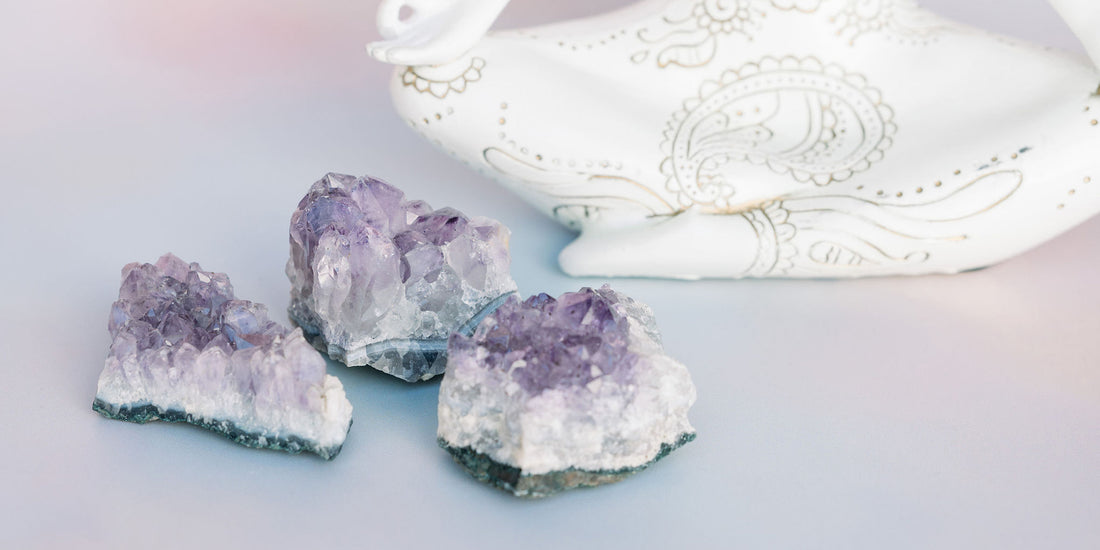This rectangular image depicts three large geode chunks positioned in the lower-left corner against a faded blue and pink background. Each geode showcases a dark, rough exterior base, succeeded by a band of white quartz, and crowned with a stunning array of amethyst crystals that transition from rich purple at the top to a lighter, almost white hue in the middle. Positioned behind these geode pieces, towards the top of the image, is a decorative white ceramic sculpture. This sculpture features gold striations and inscriptions at its base and portrays the lower half of a person sitting in a lotus position. The sculpture adds an ornamental contrast to the natural, rugged beauty of the geode pieces.